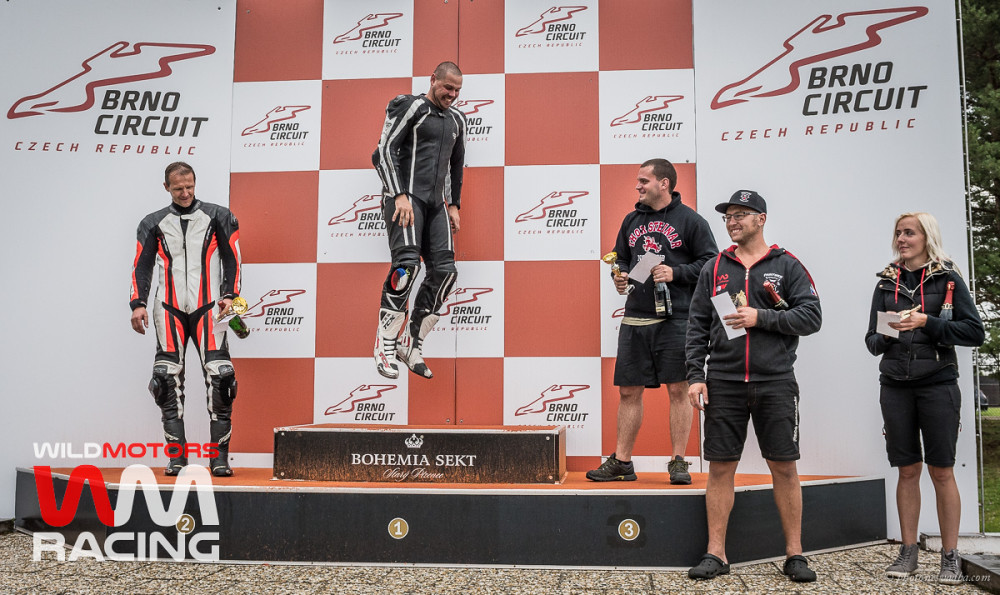The image depicts a dynamic scene at a podium award ceremony, likely held at the BRNO Circuit in the Czech Republic. Central to the image is a man who appears to be leaping or momentarily suspended in mid-air, either from a victorious jump or propelled by some device, though the exact cause is unclear. This man is situated above the highest podium spot marked with the number "1," which prominently displays the words "Bohemia Sect" in white letters.

Flanking him, two other men occupy the second and third podium positions, numbered "2" and "3" respectively. The man on the second podium is dressed in a coordinated outfit of white, black, and red, while the man on the third wears a black hoodie with red lettering and black shorts. To the right side of the image stand two additional individuals, a man and a woman, who appear to be spectators or fans. They both hold white pieces of paper and a bottle, suggesting they might be prepping for a celebratory toast.

The background features a checkerboard pattern in orange and white, interspersed with the BRNO Circuit and Czech Republic logos. In the lower left corner of the image, the text "Wild Motors" is prominently displayed in red and white, with "Racing" also visible in white letters. The scene is filled with smiling faces and a celebratory atmosphere, indicating a triumphant moment in the racing event.